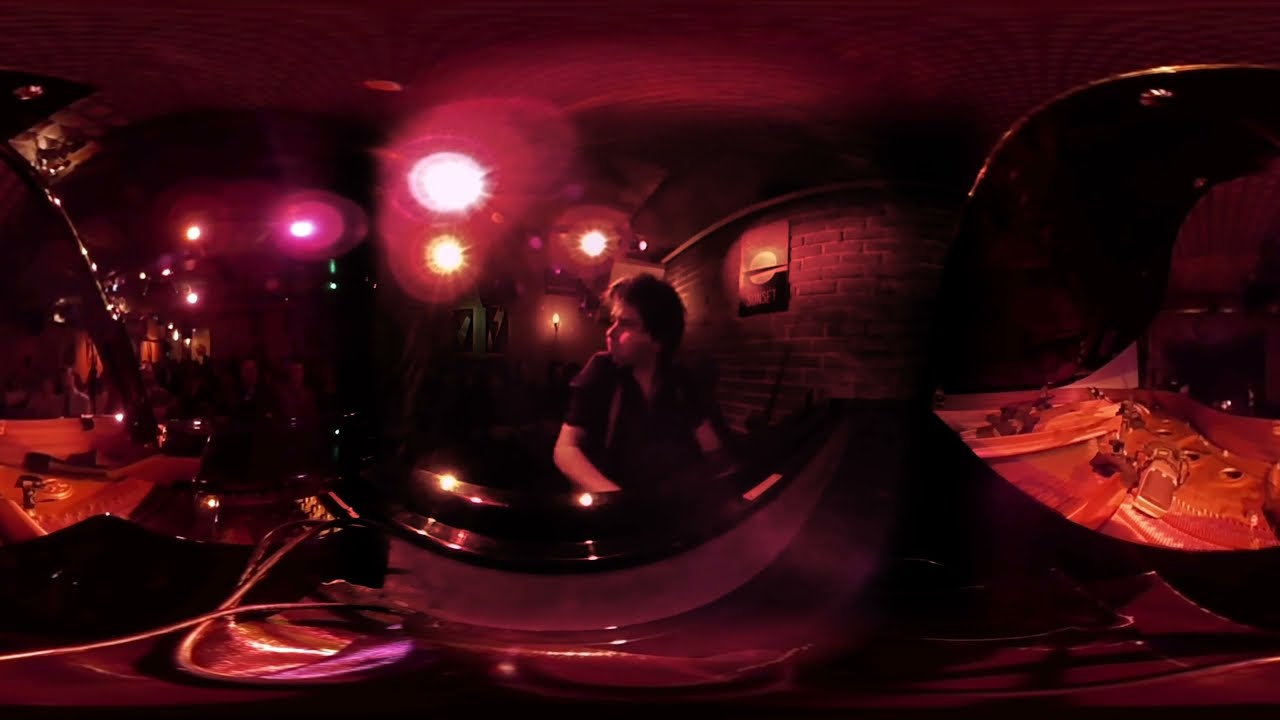The photograph captures an androgynous, white individual with puffier short black hair, seated at a piano and playing it in a dimly lit setting that resembles an intimate piano bar. The central figure, dressed in a black t-shirt, is facing to the right, deeply engaged with the piano as both their hands rest on the keys. Their mouth is open, suggesting they might be singing along while playing. The background reveals a brick wall adorned with scattered lights, casting red, orange, yellow, and green hues around the scene. The image is framed by darkness on the left and right sides, obscuring potential details. At the bottom of the image, there is a black text box with white lettering that reads "sunset" upside down, while a red text box with white letters spells out "sun side". The overall atmosphere evokes a cozy, dimly lit performance space, with the piano keys stretching prominently to the foreground and a sense of music filling the air.